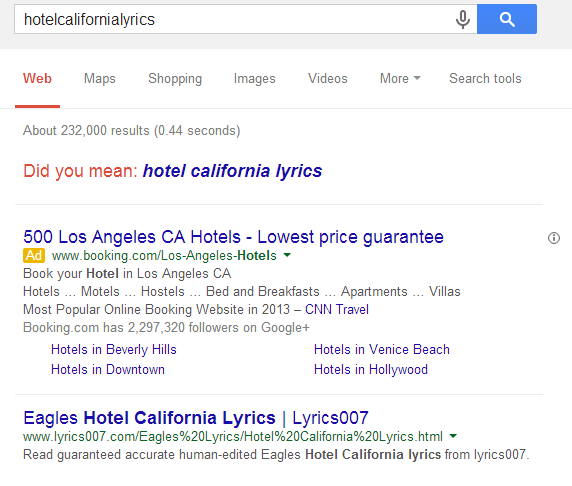The image is a horizontally rectangular screenshot of a search results page. At the top, the search bar displays a query entered without spaces: "HotelCaliforniaLyrics," creating a single, continuous string of text. To the right of the search field are the microphone and search icons. Below the search bar, a horizontal menu offers various viewing options: Web, Maps, Shopping, Images, Videos, More, and Search tools. The page indicates approximately 232,000 results with a suggestion: "Did you mean Hotel California lyrics?" The first result listed is an advertisement for "500 Los Angeles California hotels - Lowest price guarantee." Following this ad, the second listing is from Lyrics 007, titled "Eagles Hotel California lyrics." It promotes "Read guaranteed accurate human edited Eagles Hotel California lyrics from Lyrics 007."